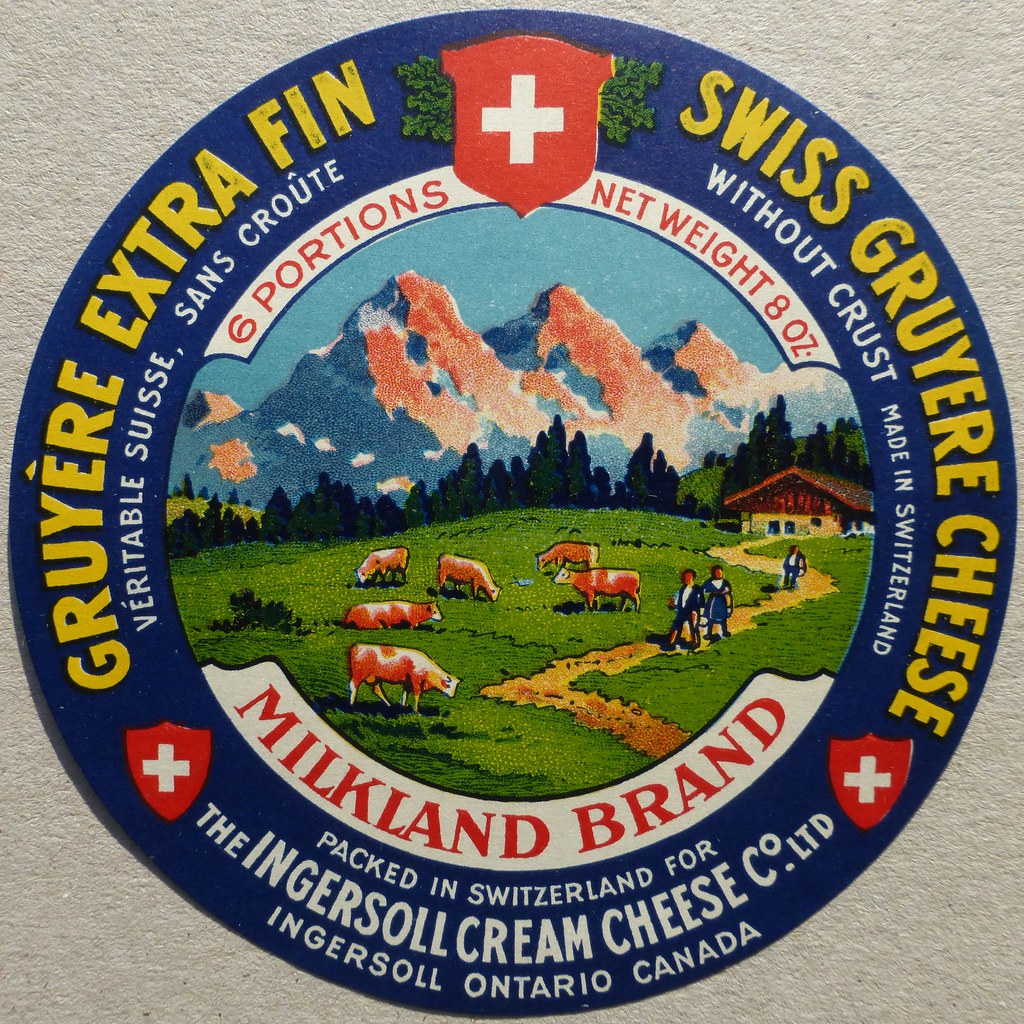The image displays a round label for Swiss Gruyere Cheese, branded by Milk Land. The background is a mottled beige, with the outer edge of the round label featuring a dark purple circle. At the top, there's a prominent red Swiss flag with a white cross. Flanking the flag, the label reads "Guyru Extra Fin" on both sides, along with some Swiss text. 

Encircling the center image, yellow text alternately spells out "Gruyere Extra Thin" and "Swiss Gruyere Cheese." A notable shield with the Swiss emblem prominently sits in the middle. Inside the circle, a digital illustration depicts a picturesque Swiss landscape, featuring the Swiss Alps, a traditional home, grazing cows, and a few Swiss people walking in the fields under a serene sky. 

At the bottom of the label, text informs that it contains six portions with a net weight of eight ounces. Essential details include the product being packed in Switzerland for the Ingersoll Cream Cheese Co. Ltd., located in Ingersoll, Ontario, Canada.